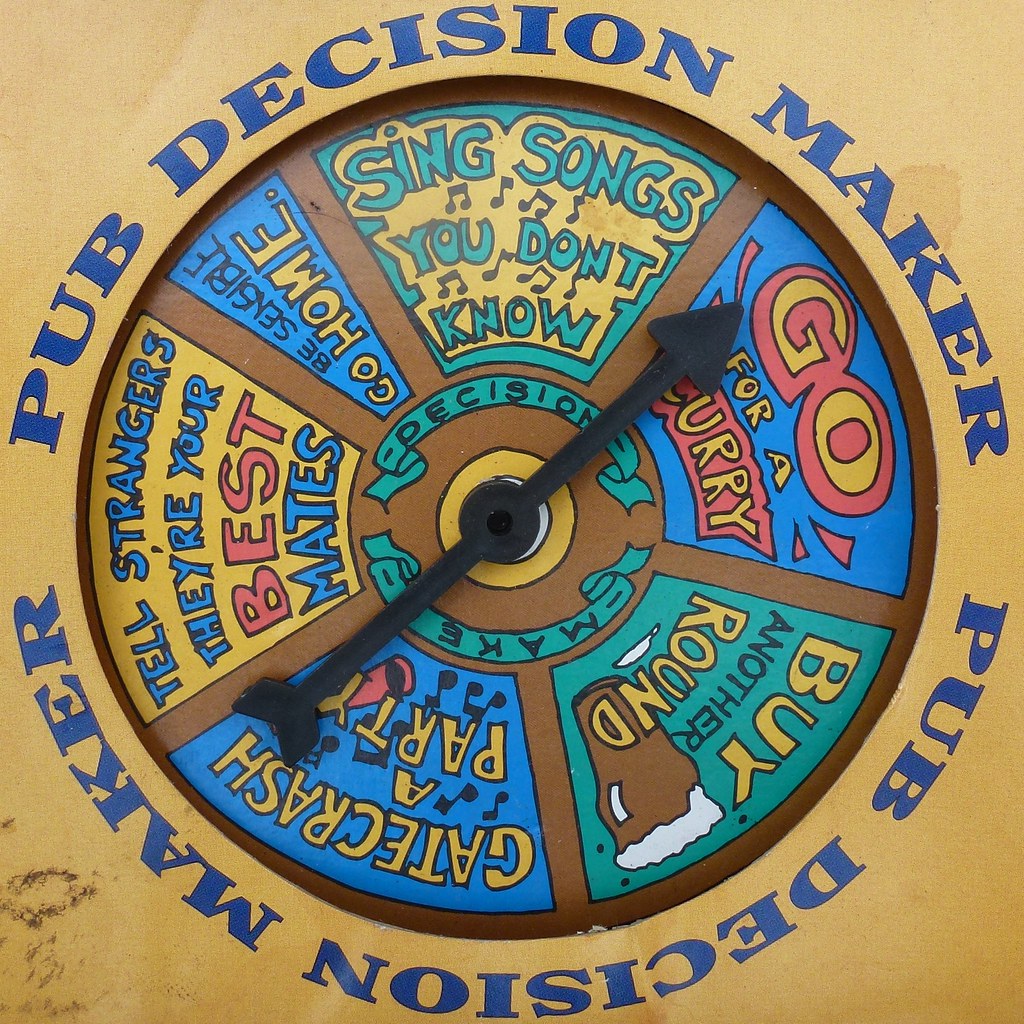The close-up image prominently features a circular device known as the "Pub Decision Maker," occupying nearly the entire frame set against a tannish brown background. The design is somewhat akin to a board game, featuring a central spinning arrow made of black plastic or rubber. This arrow points to various brightly colored and stylized sections on the disc, each representing a different playful directive for pub-goers. The options include: "Sing Songs You Don't Know," "Go for a Curry," "Buy Another Round," "Crash a Party," "Tell Strangers They're Your Best Mates," "Be Sensible," and "Go Home." The colors used are vibrant shades of blue, turquoise, yellow, red, and green, giving it a cartoonish appeal. Currently, the arrow is positioned at "Go for a Curry," inviting a humorous and spontaneous decision from its user.